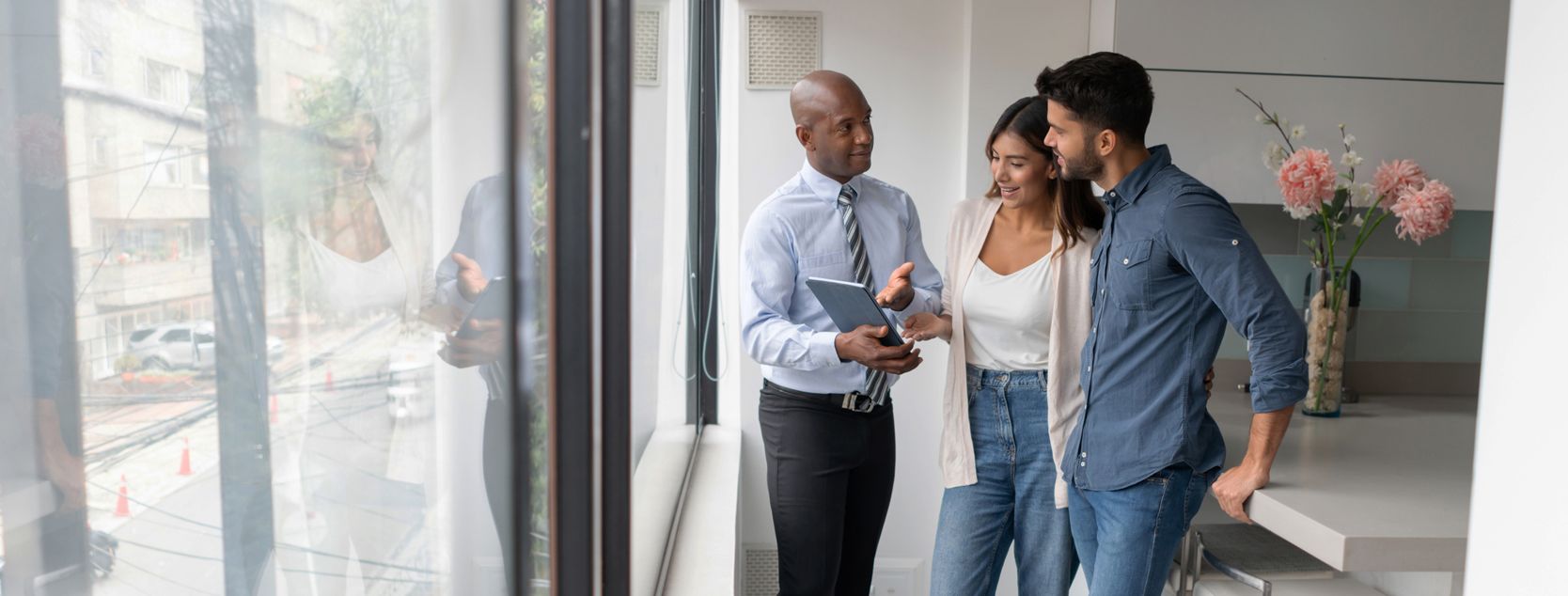In this color photograph, three adults are inside a building, standing in front of a large window that reflects their image. Outside, a busy street scene includes a parked car, road cones from recent road work, and an apartment building across the road. Inside, the scene focuses on an African American gentleman, likely a realtor, dressed smartly in a light blue dress shirt, dark form-fitting black pants, and a blue and white striped tie. He holds a tablet and is showing it to a young couple standing next to him. The woman has long dark hair, wears a light pink cardigan over a white shirt, and blue jeans. The man, with short dark hair, is dressed in a casual blue button-down shirt and blue jeans. The trio is deeply engaged in a conversation about the content on the tablet, all smiling and clearly enjoying the interaction. In the background, on a white table to their right, there is a vase containing pink flowers arranged with rocks at the base, adding a cheerful touch to the interior.